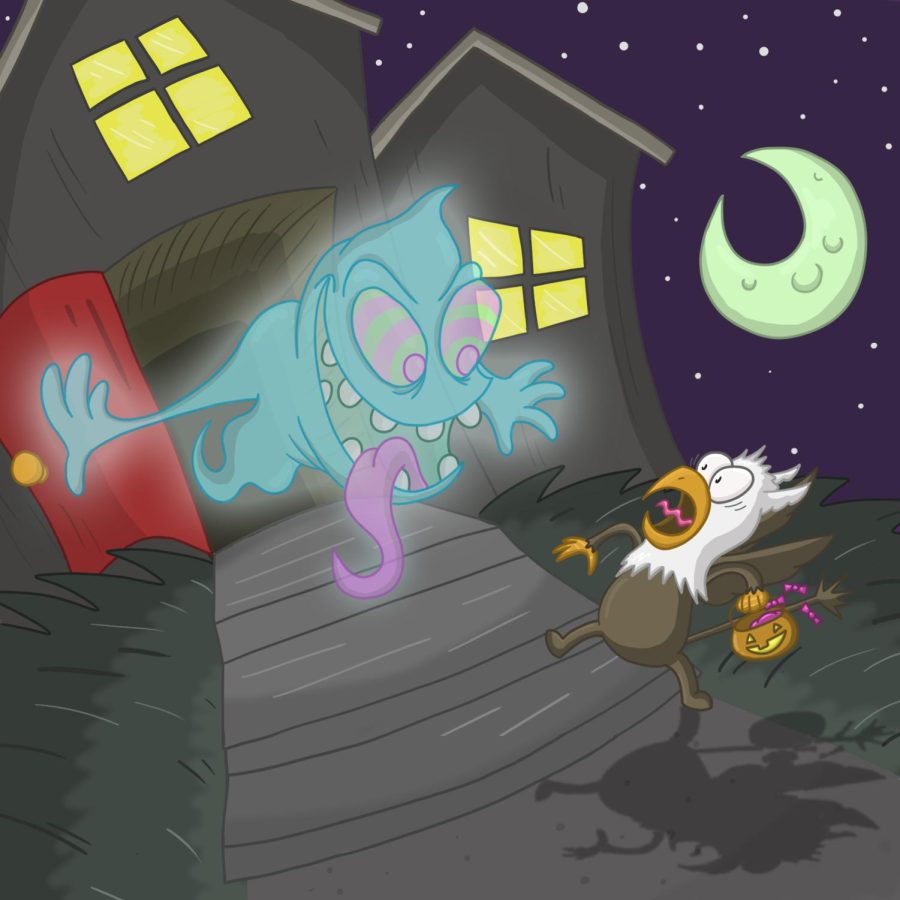The cartoon illustration depicts a dark night with a starry sky in the upper right portion and a half moon casting a light green glow. In the center of the image is a gray house with a red door and yellow-lit windows. Emerging from the door is a blue, semi-transparent ghost with jagged white teeth, a purple tongue sticking out, and eyes that are striped green and purple. Walking up the gray sidewalk towards the house, surrounded by green grass, is an anthropomorphized bird that resembles a chicken or a bald eagle. This bird has a white head, an orange beak, a brown body with legs, and is carrying a jack-o'-lantern bag filled with blue candy. The bird has a surprised expression, likely frightened by the ghost's sudden appearance, causing some of the candy to spill from the bag.